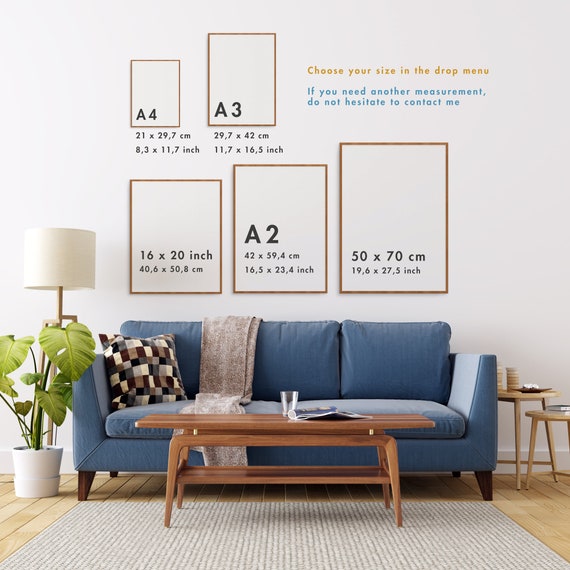This meticulously manicured living room scene showcases a blue fabric couch, which features three back cushions and two seat cushions. The couch has four stumpy brown legs and two arms, with one corner adorned by a patterned checkerboard throw pillow in various shades of black and brown. A light beige throw blanket drapes between the first and second back cushions, extending over the seat and nearly touching the floor. In front of the couch lies a modern wooden coffee table, which holds an empty glass and a rolled-up magazine. The room's light-colored hardwood flooring is partially covered by a light beige rug beneath the coffee table. To the left of the couch, a white floor lamp with a white shade stands next to a potted green house plant. On the right side, two small circular wooden end tables bear books and cups. 

The backdrop of this scene features a white wall adorned with five framed art pieces, serving as an advertisement for framing options. The text on the wall reads, "Choose your size in the drop-down menu," followed by, "If you need another measurement, do not hesitate to contact me." The displayed frames vary in size, from A4, A3, and A2, to 16 by 20 inches and 50 by 70 centimeters, with measurements indicated in both inches and centimeters beneath each frame. The frame styles include a brown framework with a white center, fitting the living room’s modern aesthetic.